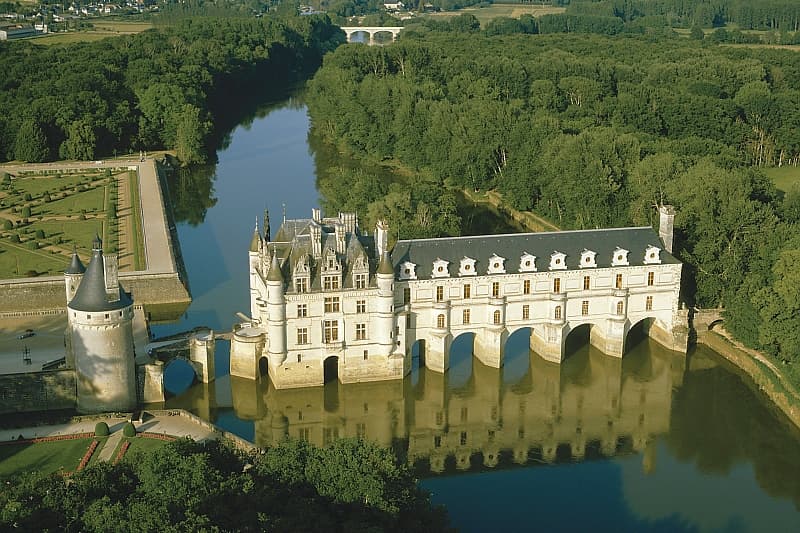The image showcases an overhead aerial view of a European-style white castle situated in the middle of a large murky brown river. This substantial structure, painted white with dark gray roofs, features at least three stories and includes arched bridges integrated into its design that allow the river water to flow through parts of the castle. The architecture highlights a considerable contrast between the castle's ornate left side, with spires and a large tower, and the more plain, elongated building on the right. Surrounding the castle, there are meticulously maintained square-shaped gardens that enhance its grandeur. Beyond the gardens on one side, a dense forest of lush green trees offers a picturesque backdrop, while in the distance, a bridge connects the landmasses on either side of the river, and a cityscape with various buildings can be seen on the horizon. The daylight illumination further accentuates the castle's beige-colored block structure, enriching the overall scenic beauty of the castle in its serene riverine setting.